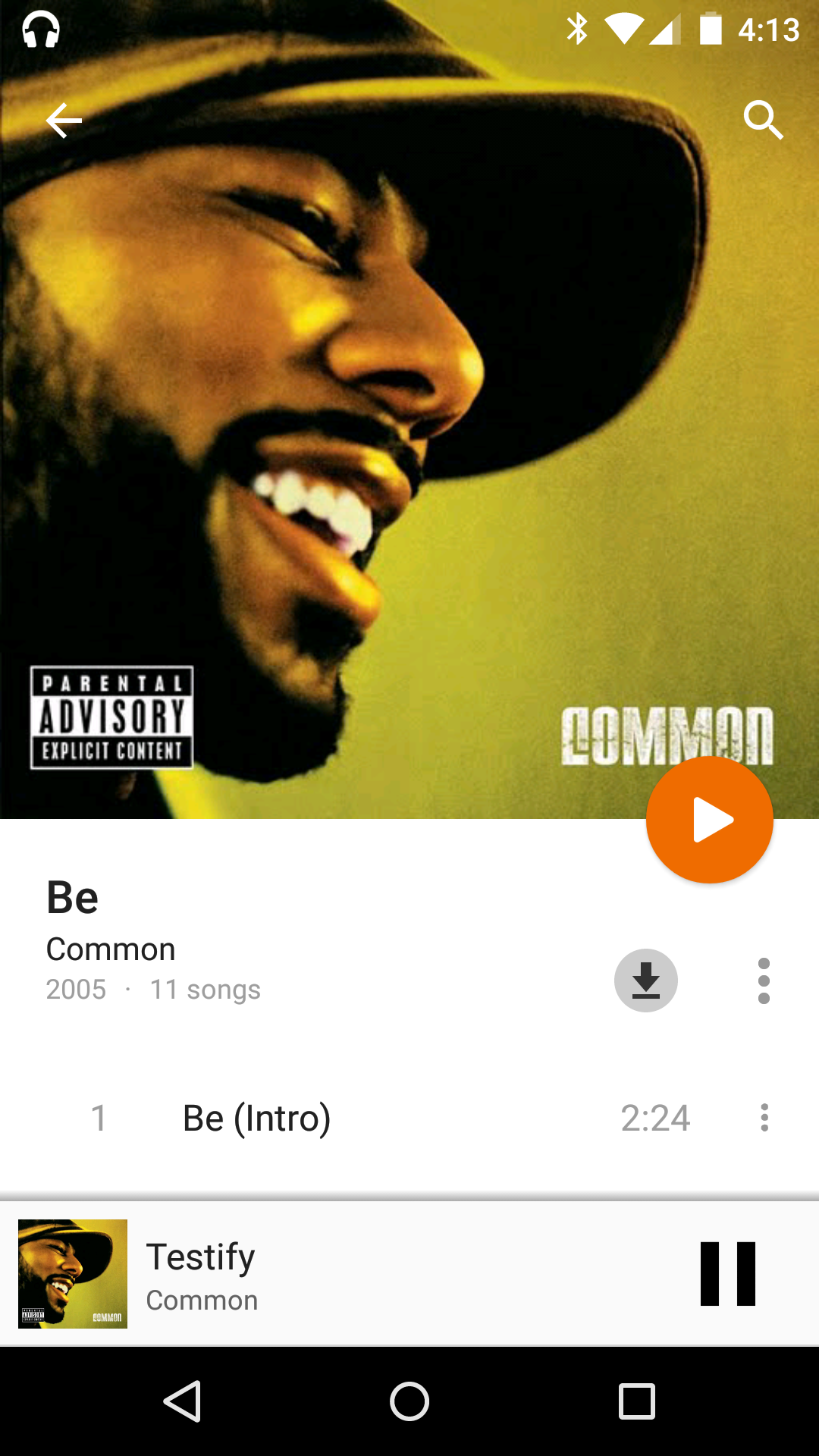The image depicts a smartphone screen showcasing a music player interface. At the top of the screen, there is an album graphic featuring a black male on the left side, laughing with his mouth open. He is wearing a brown hat and has a black mustache and beard. The background of the album art is greenish in color. To the right of the image, the word "Common" is displayed, while on the left, a black and white "Parental Advisory Explicit Content" label is visible.

Beneath the album art, there is an orange play button with a white triangle in its center. Below this play button, there's information indicating that the album is titled "Be," performed by the artist Common, released in 2005, and consisting of 11 songs. The currently playing song is "Testify," which is accompanied by a large pause button to its right. Above the currently playing song, the first track listed is "Be (Intro)" with a duration of 2 minutes and 24 seconds.

At the very bottom of the screen, there is a black border containing music control icons: a triangle pointing to the left (likely a back button), a circle, and a white square (probably the options or more settings button).